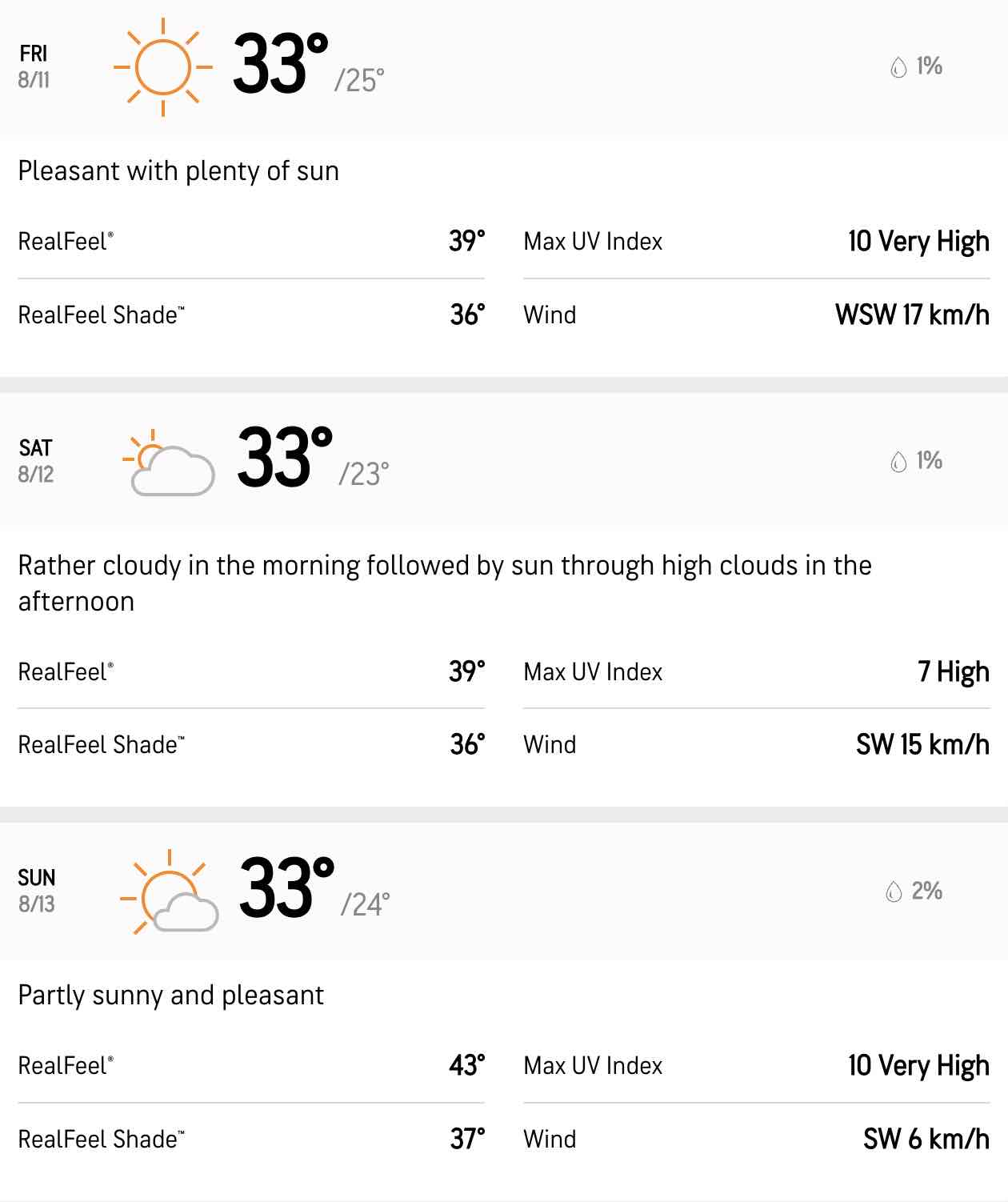A detailed weather forecast displayed on a tablet screen is segmented into three sections for three consecutive days. 

**Friday, August 11th (FRI 8\\11):**
- **Condition:** Sunny
- **Temperature:** 33°C (bold black) / 25°C (light gray)
- **Precipitation Probability:** 1% (icon: raindrop)
- **Details:** 
  - Pleasant with plenty of sun
  - Real Feel: 39°C
  - Max UV Index: 10 (Very High)
  - Real Feel in Shade: 36°C
  - Wind: WSW at 17 KM/H

**Saturday, August 12th (SAT 8-12):**
- **Condition:** Partly Cloudy with Sun
- **Temperature:** 33°C (bold black) / 23°C (light gray)
- **Precipitation Probability:** 1% (icon: raindrop)
- **Details:**
  - Rather cloudy in the morning, followed by sun through high clouds in the afternoon
  - Real Feel: 39°C
  - Max UV Index: 7 (High)
  - Real Feel in Shade: 36°C
  - Wind: SW at 15 KM/H

**Sunday, August 13th (SUN 8-13):**
- **Condition:** Partly Sunny and Pleasant
- **Temperature:** 33°C / 24°C
- **Precipitation Probability:** 2% (icon: raindrop)
- **Details:**
  - Real Feel: 43°C
  - Max UV Index: 10 (Very High)
  - Real Feel in Shade: 37°C
  - Wind: SW at 6 KM/H